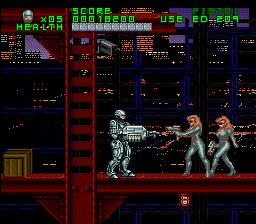Screenshot of a vintage video game featuring RoboCop, likely from the Super Nintendo era. The scene depicts RoboCop standing on a red steel girder platform with matching uprights. To his left, there's a brown cardboard box. RoboCop is holding a weapon, facing off against two women clad in green bodysuits with vivid orange hair. In the upper left corner, a HUD displays RoboCop's head alongside "TIME: 05," a gray health bar labeled "HEALTH," a score of 18,200 points, and the prompt "USE ED209."